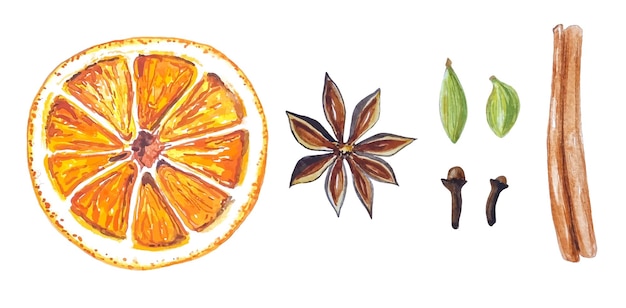The image displays a hand-drawn, rustic illustration of various spices and food items on a white background, reminiscent of watercolor or marker sketches. At the left, there's an orange, cut in half to show the juicy interior. Adjacent to the orange, there's a prominent star anise with its distinctive eight teardrop-shaped brown petals surrounding a small yellow center. Nearby are what appear to be green teardrop-shaped anise seeds or another type of aromatic seed. Below these, there are two small mushroom-like shapes, possibly cloves. Towards the right, a solitary cinnamon stick lies horizontally. The entire assortment consists of elements that could be used in creating stock images or clip art for culinary or spice-themed graphics.